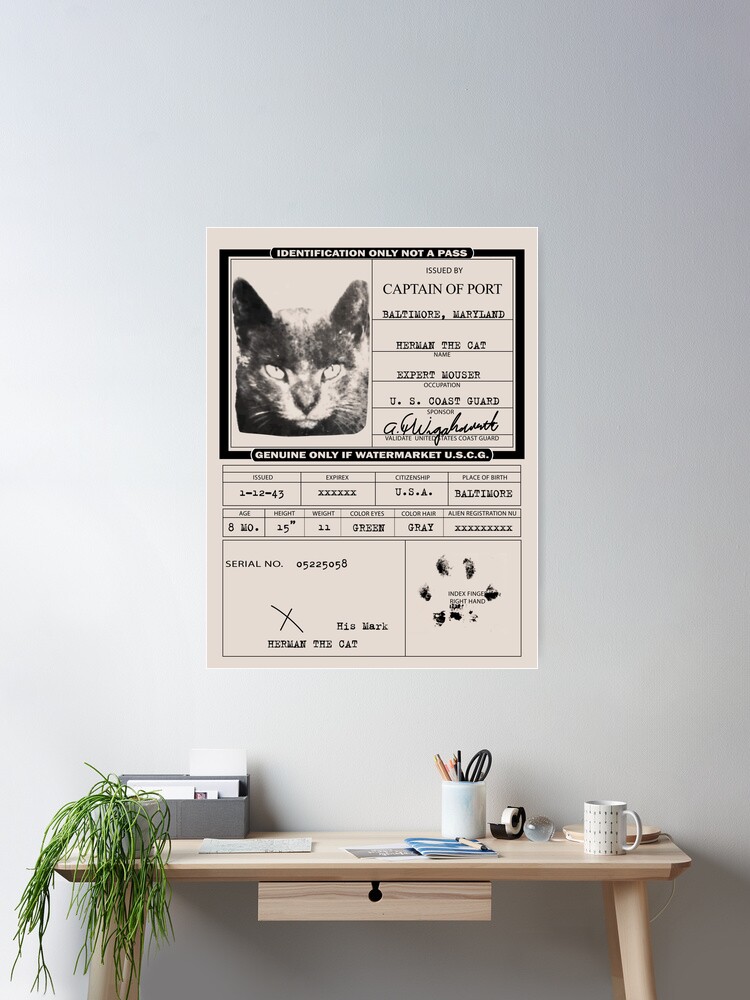The vertical image depicts a home office scene with a light wood desk situated against a gradient gray and white wall. Dominating the wall above the desk is a light tan poster outlined in black, resembling an ID card. This poster features a mean-looking black and white cat with a serious expression in the top-left quadrant and the title "Captain of Port Baltimore, Maryland" to the right. Beneath the cat's picture, the ID card details include the name "Herman the Cat," occupation "Expert Mouser," and sponsor "U.S. Coast Guard." Additional information includes a serial number, a paw print, and further specifics like Herman's age, height, and weight.

On the desk itself, a variety of items are neatly arranged. A small green plant cascades over the left corner next to a stationery box filled with assorted letters and papers. Scattered across the desk are some papers and notebooks, a white pencil holder containing pens and pencils, and a cup of coffee with a dotted design. Also present are a tape dispenser, a small clear paperweight, and a white desk lamp positioned behind the coffee cup. The desk features a single drawer in the center, adorned with a lock symbol.